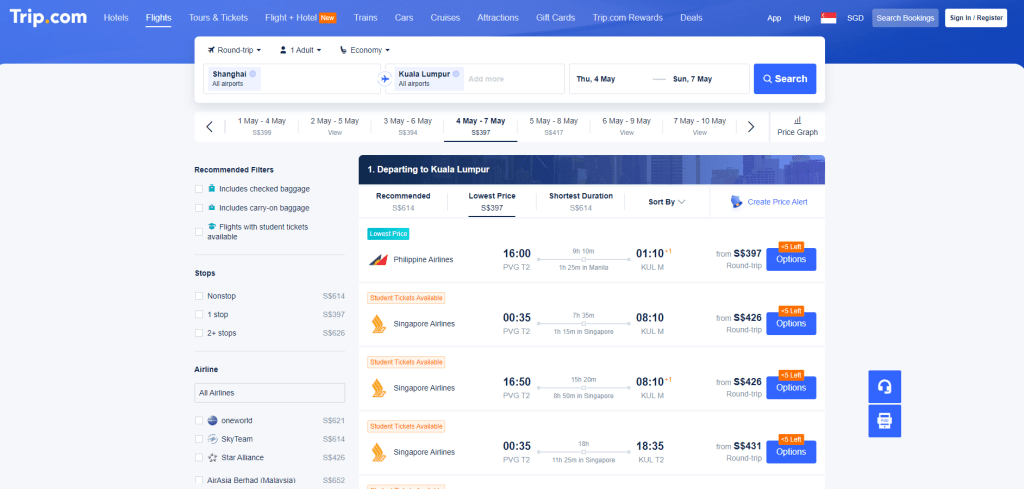**Detailed Caption:**

This is a detailed screenshot of the Trip.com website. In the upper left corner, the site’s logo, "trip.com," is prominently displayed. The main section of the webpage features various flight options and essential travel information. 

At the top of the interface, you can see the selected travel route: "Shanghai (All Airports)" and "Kuala Lumpur (All Airports)," along with the travel dates, specified as "Thursday, 4 May through Sunday, 7 May." Directly beneath this, alternative date ranges are listed: "1 May to 4 May," "2 May to 5 May," "3 May to 6 May," and "4 May to 7 May" — the last of which is highlighted.

Further down, a summary line reads "One departing to Kuala Lumpur recommended," followed by various flight details such as "Lowest price," "Shortest duration," and respective prices indicated. A distinct blue button displays the lowest price with Philippine Airlines offering a round trip from "1600 to 110," priced at the lowest rate, with a note that there are only "five left."

Additionally, there are several rows dedicated to student ticket options with Singapore Airlines, each showing different departure and arrival times, ticket prices, and an "Options" button for further choices. These entries repeat in the following pattern: "Student tickets available, Singapore Airlines," including the specific departure and arrival times and the associated prices.